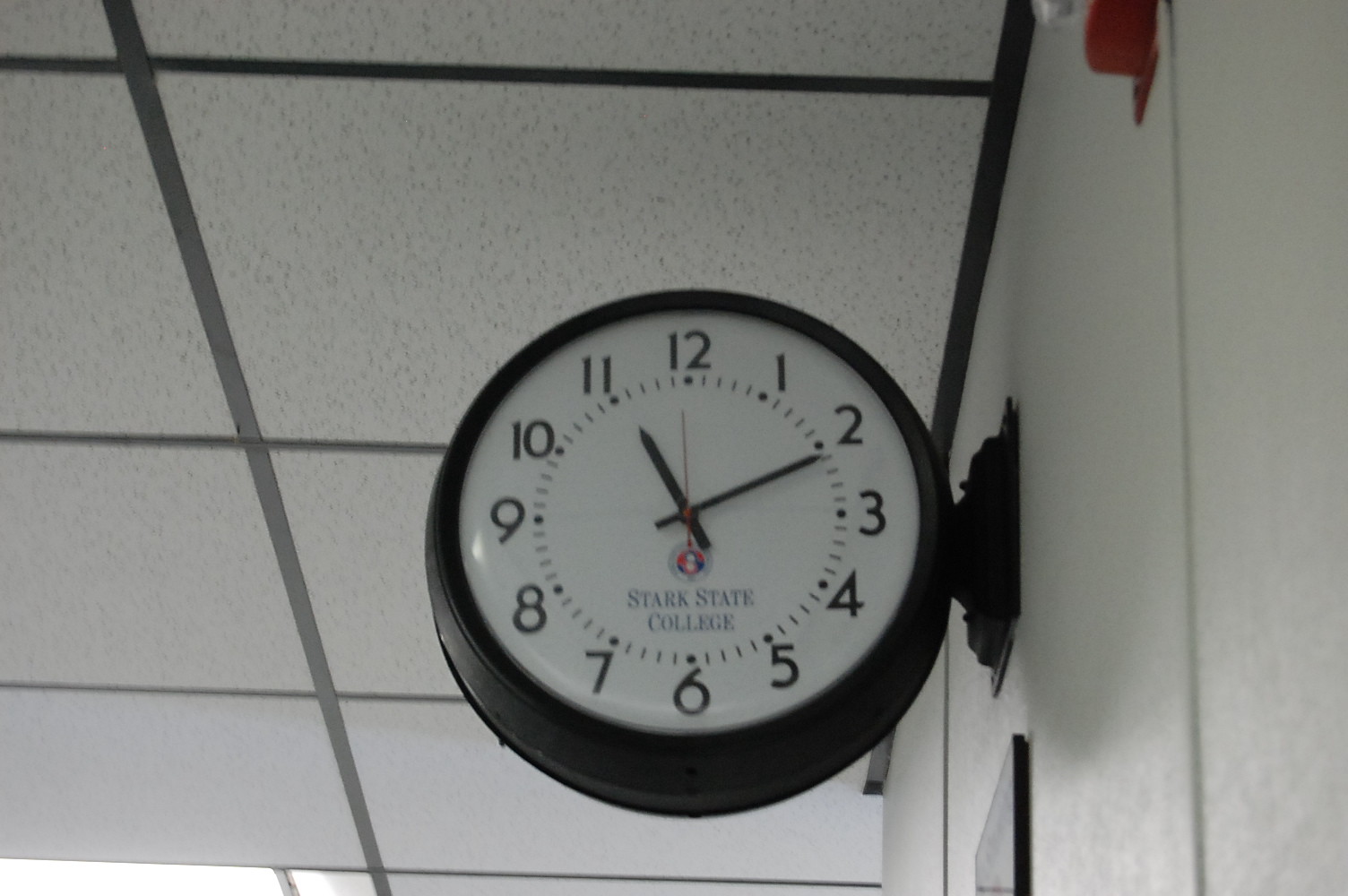The photograph showcases a round clock mounted on a wall at Stark State College. The clock features a black housing and a white face with black numbers (1-12) and black hands, with a red second hand. The time displayed is 11:11 and 59 seconds. Below the hands, "Stark State College" is inscribed, indicating the location. The clock is attached to the wall with a black base. The background reveals a white wall with a small, red fire alarm located in the upper right corner. The ceiling is composed of white acoustic tiles set in a metal framework, and a single fluorescent light is visible in the bottom left corner of the image. The clock appears to be double-sided and is possibly located within a classroom or similar academic setting.